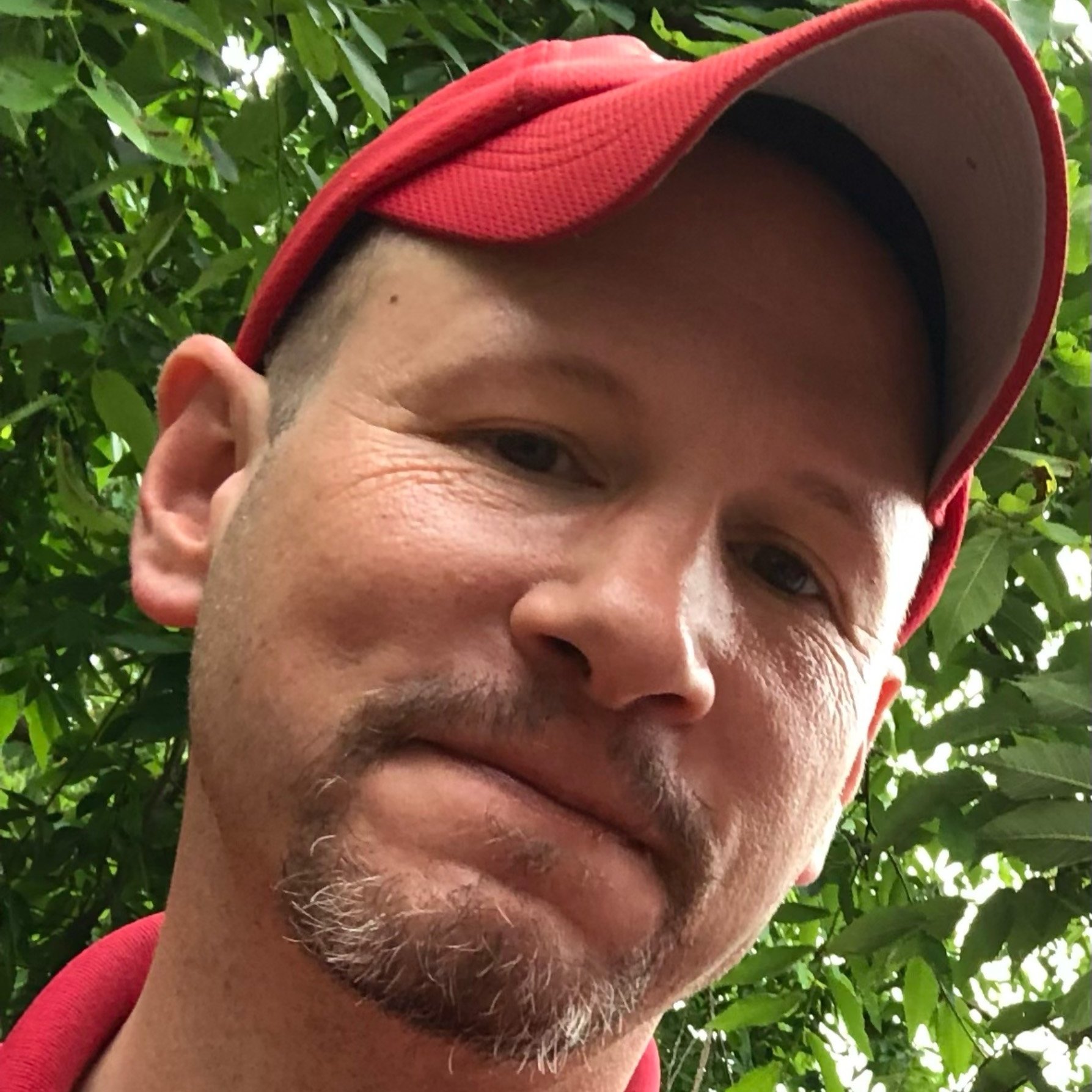This close-up selfie captures a Caucasian man with a warm smile and pursed lips, giving a slight dimple in his cheek. He wears a red baseball cap and a red T-shirt, the collar just visible. His short, neatly trimmed hair frames a face with brown eyes and subtle facial hair comprising a goatee and mustache, interspersed with a few grey strands. Wrinkles adorn the areas around his eyes, hinting at his late 30s. The man stands slightly diagonally, looking directly at the camera against a backdrop of dark green leaves and almost black branches, possibly in a natural outdoor setting. His smooth, light complexion, coupled with his relaxed facial expression and slight downward gaze, suggests a casual, unposed moment.